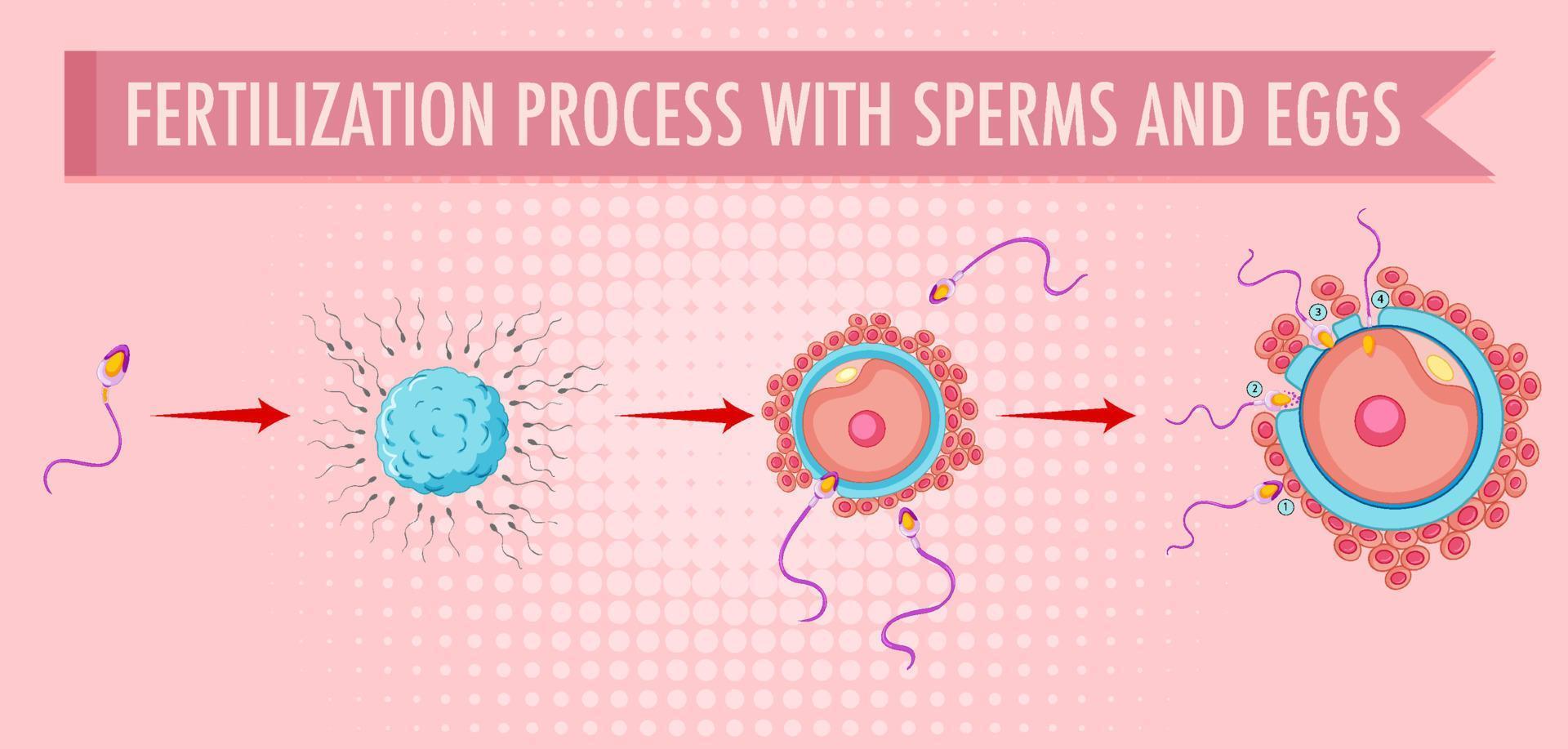The image is an educational diagram illustrating the fertilization process, set against a pink background. At the top, a dark pink banner with white, capitalized text reads "FERTILIZATION PROCESS WITH SPERMS AND EGGS." On the far left of the image, a singular sperm with a purple head and tail is highlighted. A red arrow directs attention to a blue egg that is being approached by multiple grey sperms. Another red arrow points to the subsequent stage where a sperm is penetrating the egg. The final part of the diagram shows the process of insemination with four sperms surrounding the egg, and the initial stages of cell division.